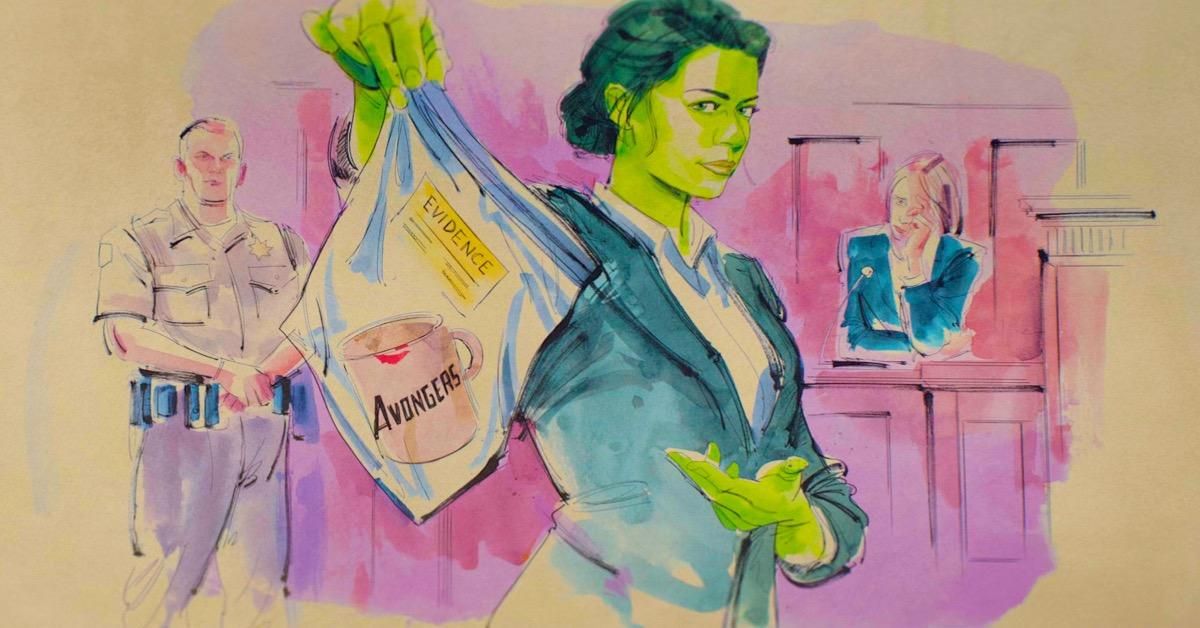In this detailed watercolor illustration of a courtroom, the central figure is a woman with greenish skin, hair styled in a dark bun, wearing a tailored black suit and white shirt. She appears to be an attorney and is holding up a plastic evidence bag with a yellow sticker labeled "evidence." Inside the bag, there is a pink mug with black writing that seems to spell "Avongers," along with a noticeable red lipstick mark on the rim. A police officer or bailiff in a gray uniform stands on the left side, hands folded, exuding a serious demeanor. To the right and slightly behind the attorney, another woman, dressed in a blue shirt, sits with her face buried in her hands, seemingly distressed. The scene includes an array of colors such as black, white, gray, various shades of blue, and pink, and the overall artwork showcases a skilled artist's depiction of a tense courtroom moment.